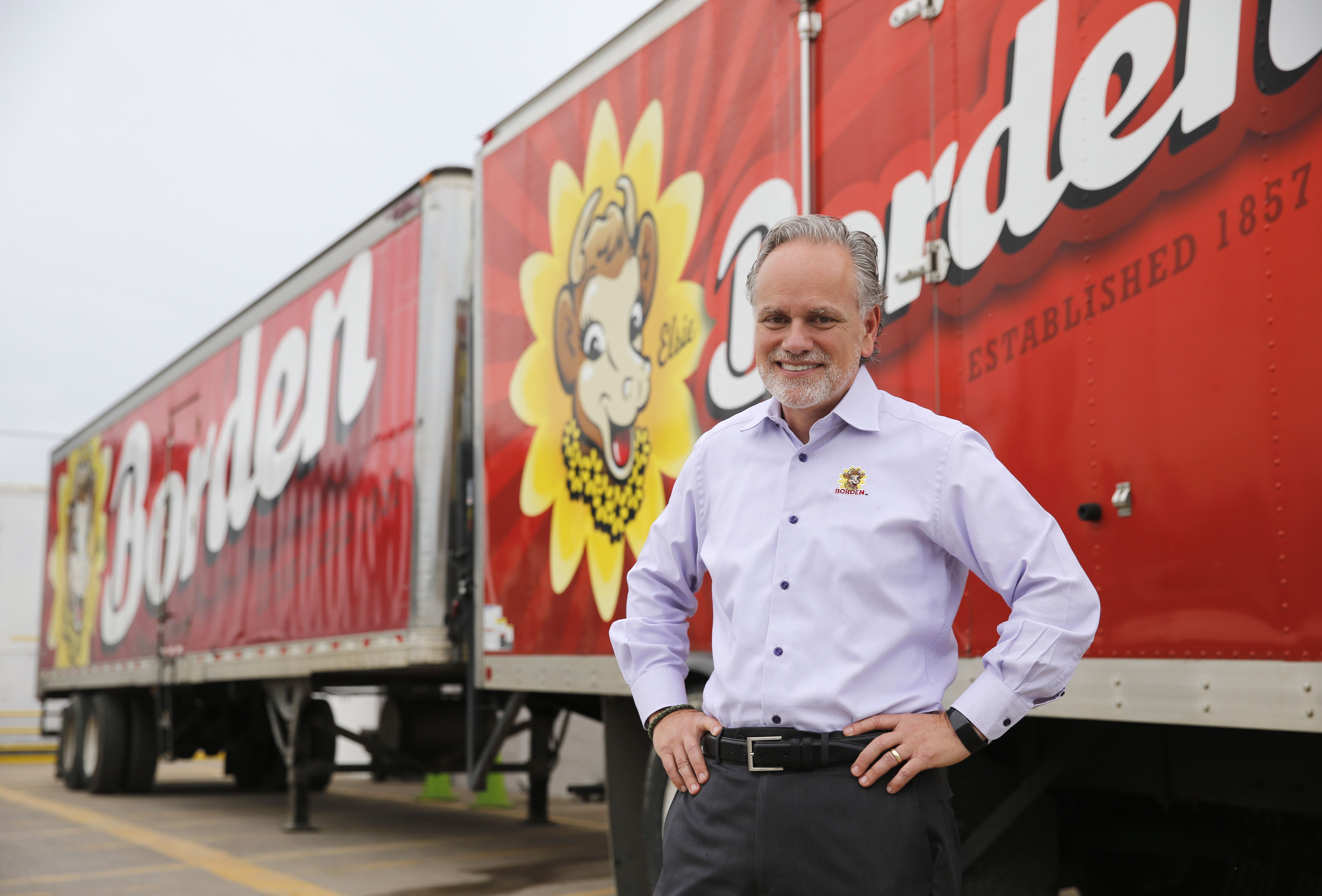This outdoor photograph captures a white man with a high forehead, gray hair, and a short gray beard. He sports a white shirt emblazoned with the emblem of Elsie the Borden cow, an image of a cow surrounded by a daisy-like flower, and the word "Borden." He also wears blue jeans with a black belt and a silver buckle. On one arm, he has a watch, possibly a Fitbit, and he is adorned with a wedding ring. The man stands confidently with his hands on his hips, smiling at the camera. Behind him are two large red trailers, side by side, displaying the Borden logo and the text "Established 1857." These trailers, which are parked with their jacks down, prominently feature the iconic smiling cow, Elsie, who is adorned with a yellow lei. The overall atmosphere is somewhat subdued, indicated by the overcast sky.